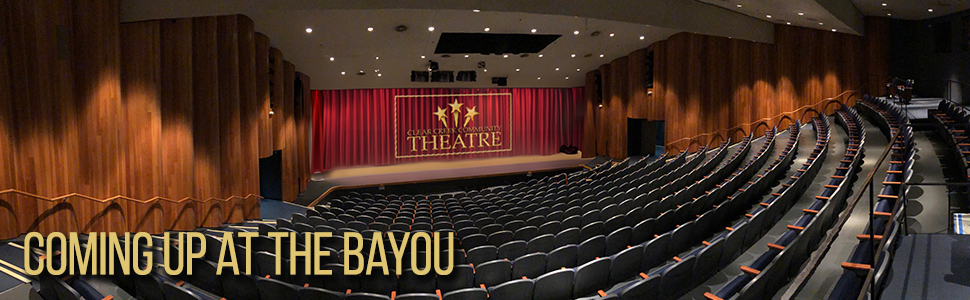This is a panoramic advertisement photograph for Clear Creek Community Theater, likely intended for a website or social media. The image captures a long, narrow, landscape-style interior view of an empty, circular-shaped theater. The seats are an array of deep blue to black shades with traditional wooden armrests, arranged in descending rows between brown wooden-paneled walls. In the bottom background of the photo is the stage, adorned with a red curtain featuring text that reads, "Clear Creek Community Theater," flanked by three gold stars. Additional features include gray flooring and ceiling lights that illuminate the space. In the bottom left corner of the image, overlaid in gold capital letters, is the promotional text, "COMING UP AT THE BAYOU." The theater also includes accessible seating areas with entrances and exits at the ends of the stage.